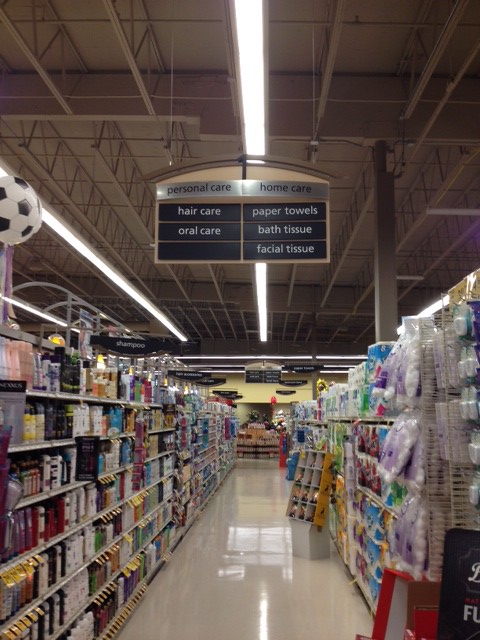The image depicts a store aisle with a sign overhead designating it as "Personal Care," with subcategories including "Hair Care" and "Oral Care." Adjacent to this, another column is labeled "Home Care," listing items such as paper towels, bath tissues, and facial tissues. Shelves on both sides of the aisle are stocked with various products corresponding to these categories. The floor is either tiled or painted with a glossy finish that reflects the overhead lighting. The ceiling features a truss-based structure, with parallel trusses running along the aisle and perpendicular supports intersecting them. A structural pole support is visible on the right-hand side of the aisle. In the distance, a section bathed in a pinkish hue suggests the presence of another store area, potentially a deli, though it remains out of focus.